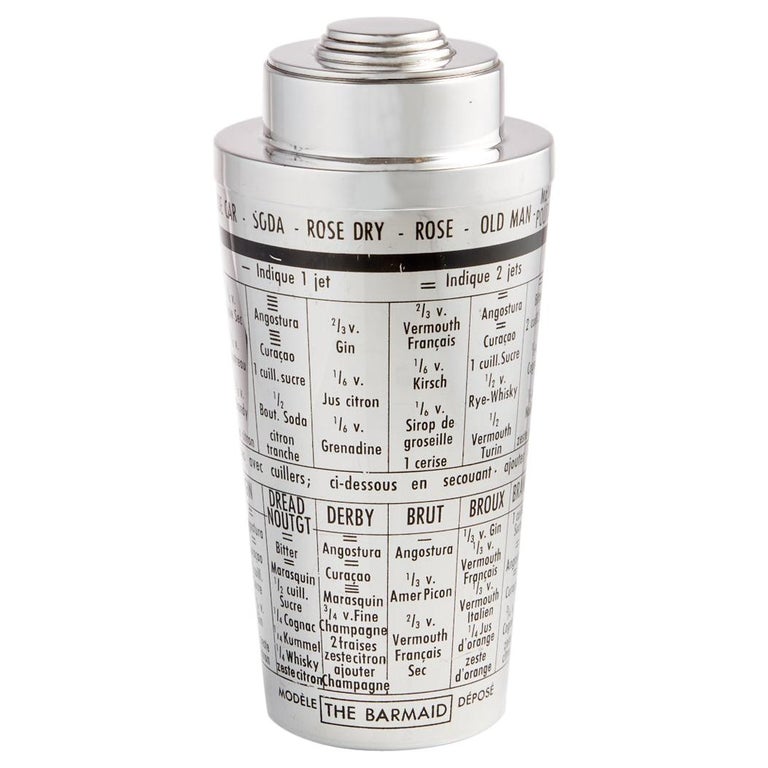The image depicts a vintage bartender's tool, specifically a cocktail shaker made of either aluminum or chrome, with a sleek, metallic finish. Set against a plain white background, the shaker is the sole focus and features black lettering printed around its surface. The bottom of the shaker is marked with the inscription "Model the Barmaid de Posay," while the top section is adorned with a band listing various cocktail ingredients in a foreign language, including "Soda," "Rosé Dry," "Rosé Old Man," and others. The cylindrical body of the shaker displays intricate recipes for a variety of cocktails, such as:

- A recipe involving two-thirds vermouth, a quarter measure of kirsch, and an eighth measure of syrup de graciel, garnished with a cerise.
- A "Derby" cocktail consisting of Angostura, Curacao, Maraschino, three-quarters measure of fine champagne, and two fraises.
- A "Dreadnought" recipe, which is less clear but includes elements such as Brut or Broux.

Further instructions for cocktails include ingredients like gin, citron juice, and grenadine. Though the exact quantities and some terms are partially obscured or difficult to decipher, the shaker serves as a comprehensive guide for mixing a variety of vintage alcoholic beverages.